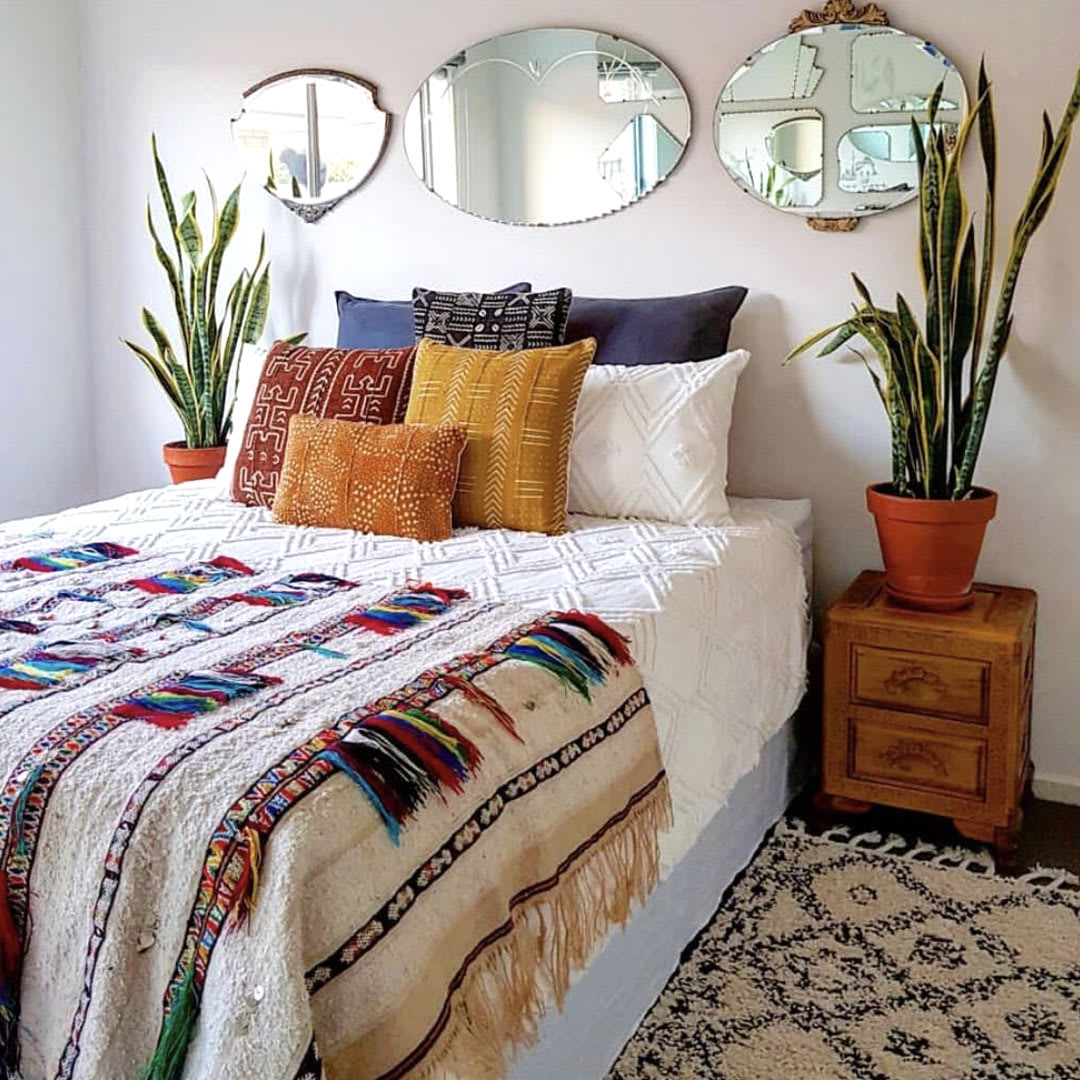The photograph depicts a bright, daytime scene of a neatly arranged bedroom interior. The camera focuses on a wall that meets another at the upper left corner of the image, capturing a portion of both walls. A bed, aligned with the main wall, extends into the room with its head positioned against the wall. The bed features a white knitted bedspread with a raised diamond pattern, partially covered at the foot by a multicolored blanket. This blanket is light brown with hanging fringe and vertical rows of color including red, white, brown, blue, and green. 

At the head of the bed, a variety of throw pillows in different colors are arranged. Behind the pillows, there are three circular mirrors mounted on the otherwise light-colored wall, reflecting the room's natural daylight. Blue pillows are placed at the back with a black and white one in the center. The front row of pillows consists of a red and white pillow, a yellow and white pillow, a plain white pillow, and a small dark orange one.

On either side of the bed, tall potted plants add a touch of greenery to the room. The plant on the right sits atop a small brown nightstand, while the plant on the left is presumed to be on a symmetrical nightstand, though it's not visible in the frame. The overall atmosphere of the room is bright and clear, with ample natural lighting enhancing the clarity of the image.